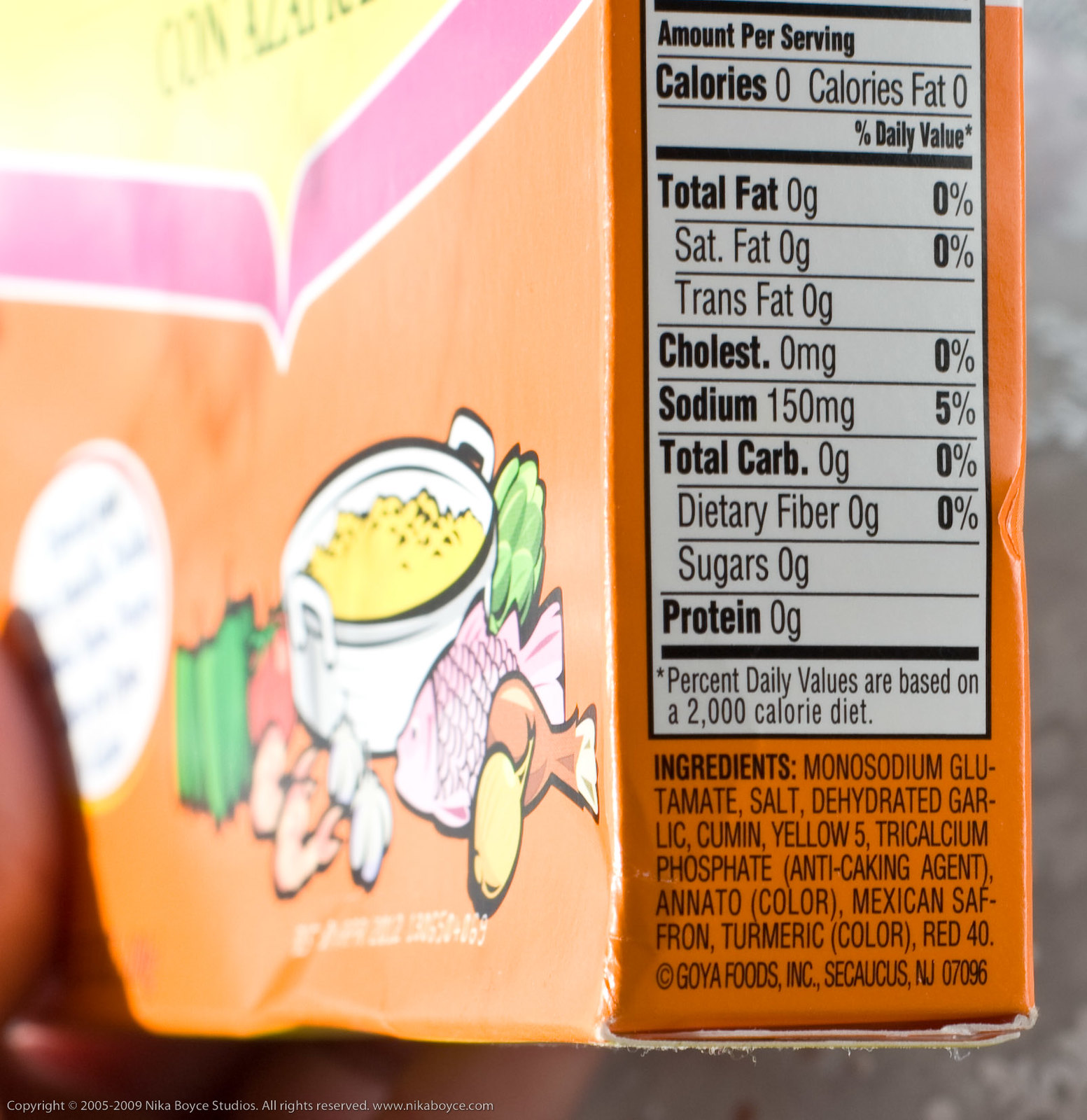This is a close-up photograph of the side of a predominantly orange cardboard food container, likely a cereal box, prominently displaying the nutritional facts. The white rectangle with black text reveals that per serving, the product contains 0 calories, 0 calories from fat, 0 grams of total fat, 0 grams of saturated fat, 0 grams of trans fat, 0 milligrams of cholesterol, 150 milligrams of sodium (5% of the daily value), 0 grams of total carbohydrates, 0 grams of dietary fiber, 0 grams of sugars, and 0 grams of protein. A small asterisk indicates that the percent daily values are based on a 2000-calorie diet. To the left of the nutritional label, a light-skinned thumb is visible, holding the rectangular box. The bottom right side of the box features a colorful cartoon graphic depicting food items such as a fish, an onion, some greens, shrimp, and a silver pot containing yellow food. An orange background and the presence of detailed ingredients like monosodium glutamate, salt, dehydrated garlic, and cumin further complete the design.